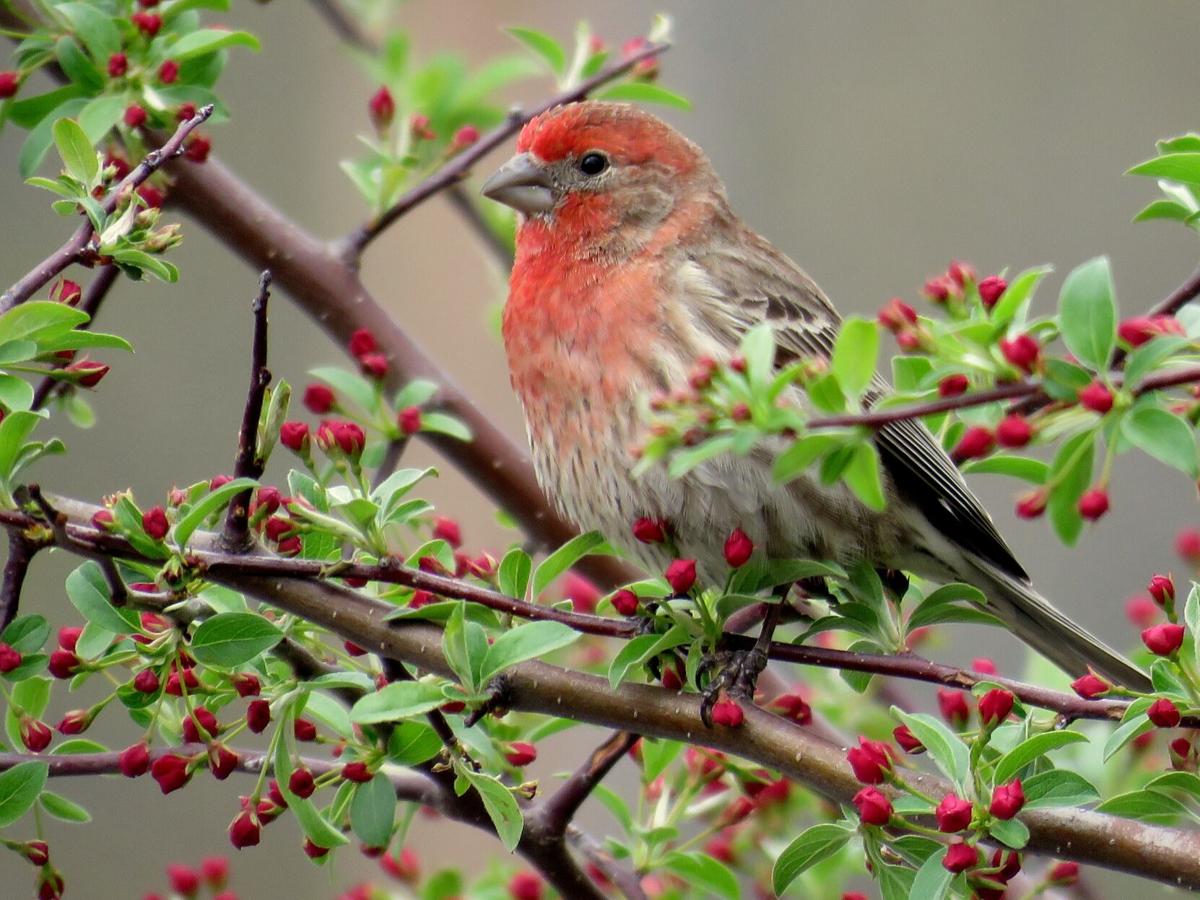The image captures a close-up of a small, distinct bird perched on a slender tree branch, surrounded by vibrant red berries and lush green leaves. The bird, predominantly gray with a subtle red-orange or pink hue on its head and chest, has striking black eyes and a short gray beak. Its tail feathers are entirely gray. The background features a soft, blurry blend of gray and red tones, suggesting the photograph was taken outdoors during the daytime with a long lens. The scene is detailed, highlighting the delicate red buds and the bird's unique coloring and serene roosting posture.